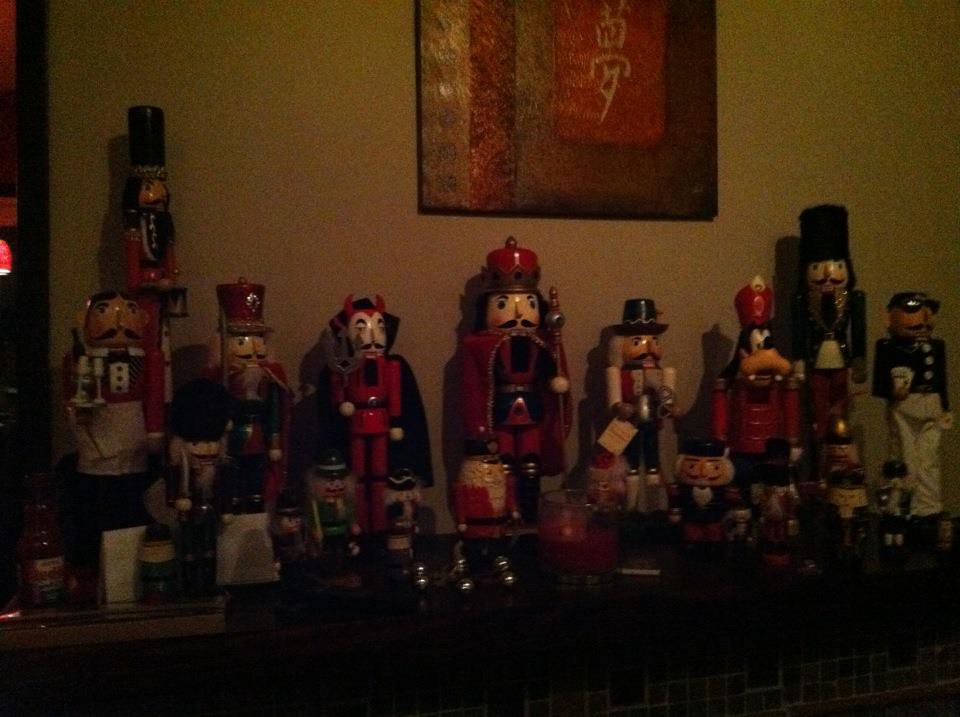This low-quality colour photograph captures the interior of a living room, specifically focusing on a mantelpiece adorned with a diverse collection of nutcrackers. Spanning from left to right in front of a dark yellow wall, the nutcrackers range in both height and design, embodying traditional Christmas soldier types with moustaches, red outfits, and distinctive hats. Among the more conventional figures are unique designs, including a devil with red horns, an orthodox-style priest with a bishop hat, a musketeer, an 1800s-era Russian soldier, a king with a crown, a leprechaun, and Goofy from Disney. The nutcrackers stand in front of a portrait-style artwork that extends beyond the frame, partially cut off. At the forefront, a smaller, even less discernible row of nutcrackers can be seen, blurred and obscured by shadows. The mantel also features additional items such as a candle, a tray with various sauces, and another smaller nutcracker. Overall, the detailed display of nutcrackers brings to mind scenes from "The Nutcracker" ballet, creating a whimsical and festive atmosphere despite the image's poor quality and limited lighting.